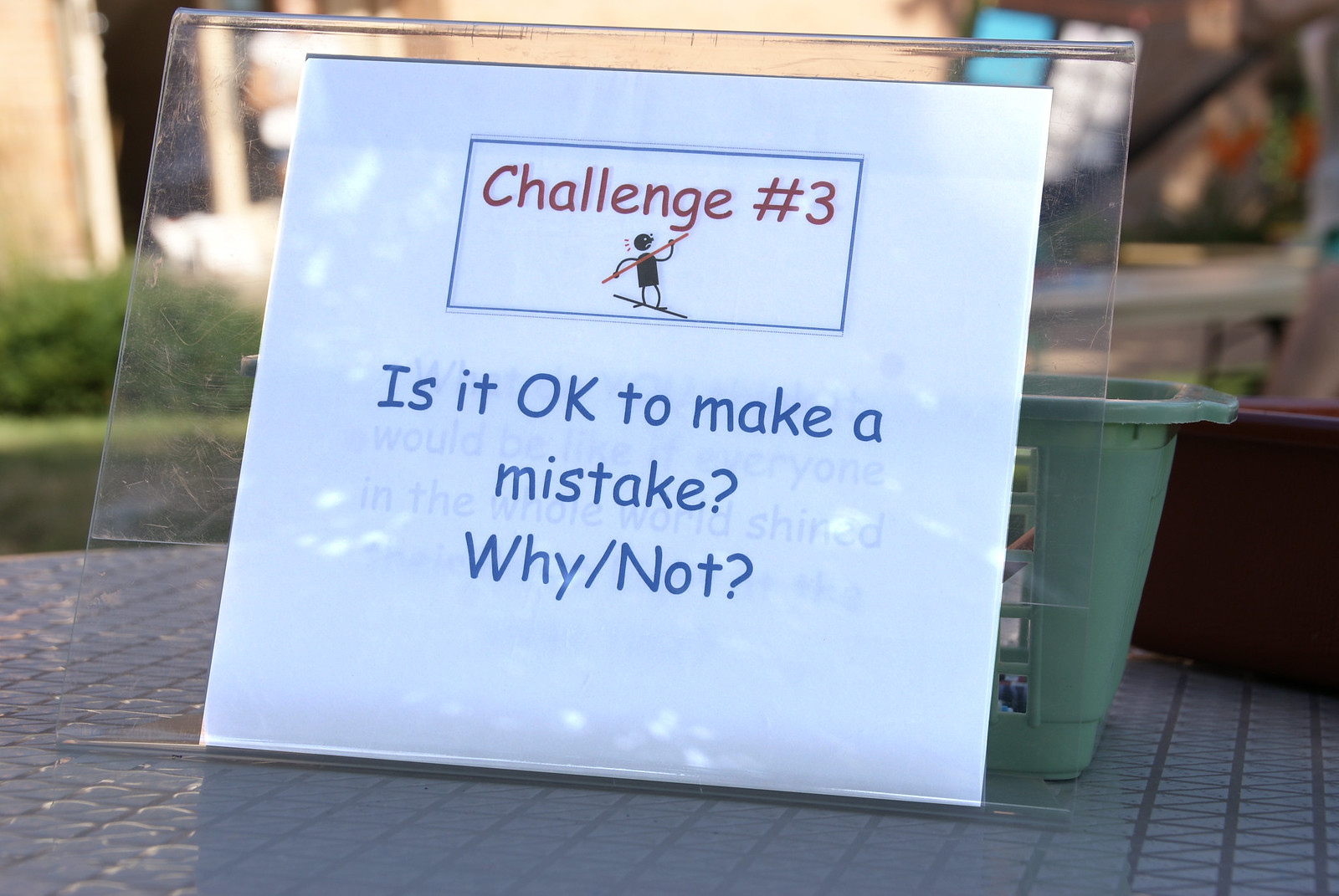The image features a textured gray table with a distinct V-pattern surface, situated outdoors. On the table is a white plastic sign holder in a V shape, containing a white sheet of paper with blue and red lettering. At the top of the paper, within a blue-outlined rectangle, it reads "Challenge No. 3" in red text. Below this, a stick figure is depicted standing on a black line, holding a large red pole across its chest with both hands. Further down, the blue text asks, "Is it okay to make a mistake? Why/Not?" Positioned behind the sign is a small lime green basket, and a dark red container is visible further back. The blurred background showcases green grass, a darker green bush, a stone building, and another table. Additionally, a person can be faintly seen exiting the building.